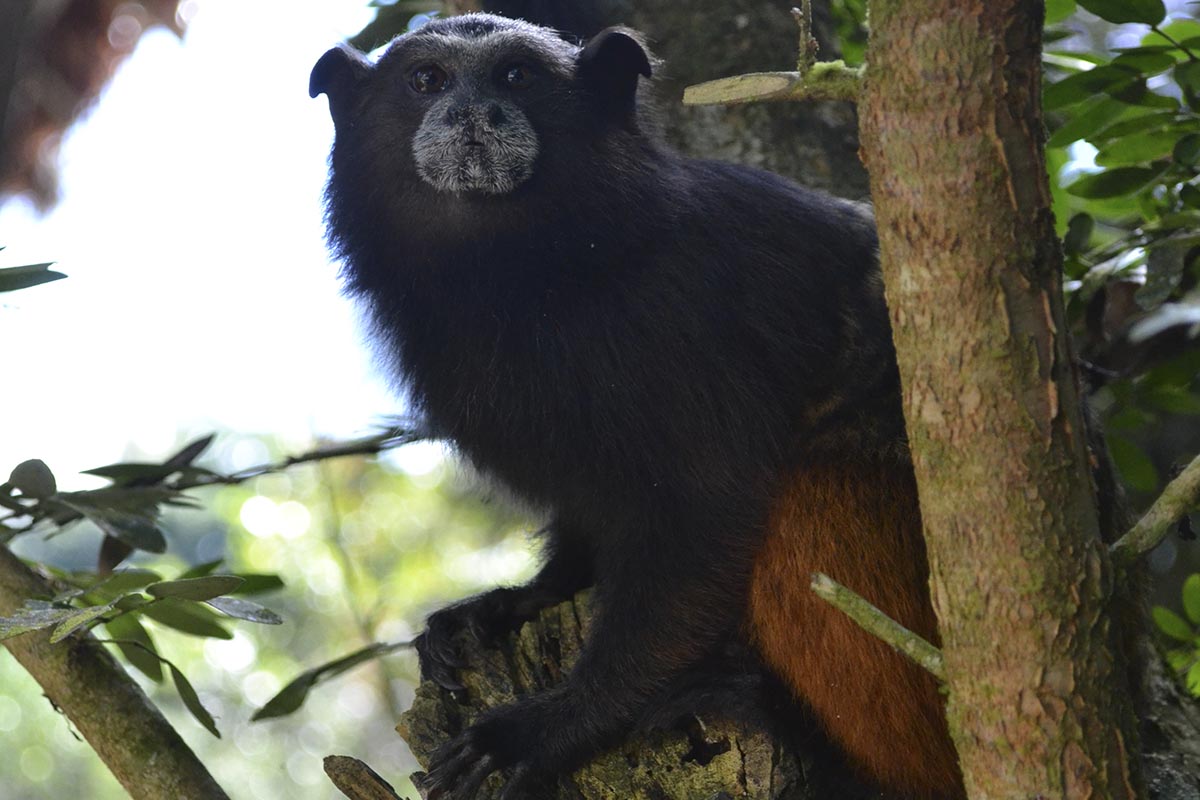Perched high in the branches of a tree, an enigmatic black-furred animal with a flattened head surveys its surroundings. Tiny ears protrude from its sides, while a circular snout and black eyes give its face a somewhat flattened appearance. With no prominent neck, its fur flows seamlessly into a stocky body supported by medium-sized arms ending in claws. The animal's legs are brownish in color and it is squatting comfortably, hugging a tree stump with one paw while balancing on a tree branch. Lush green leaves surround the creature, and bright sunlight filters through the foliage, creating a stark contrast of light and shadow in the scene.